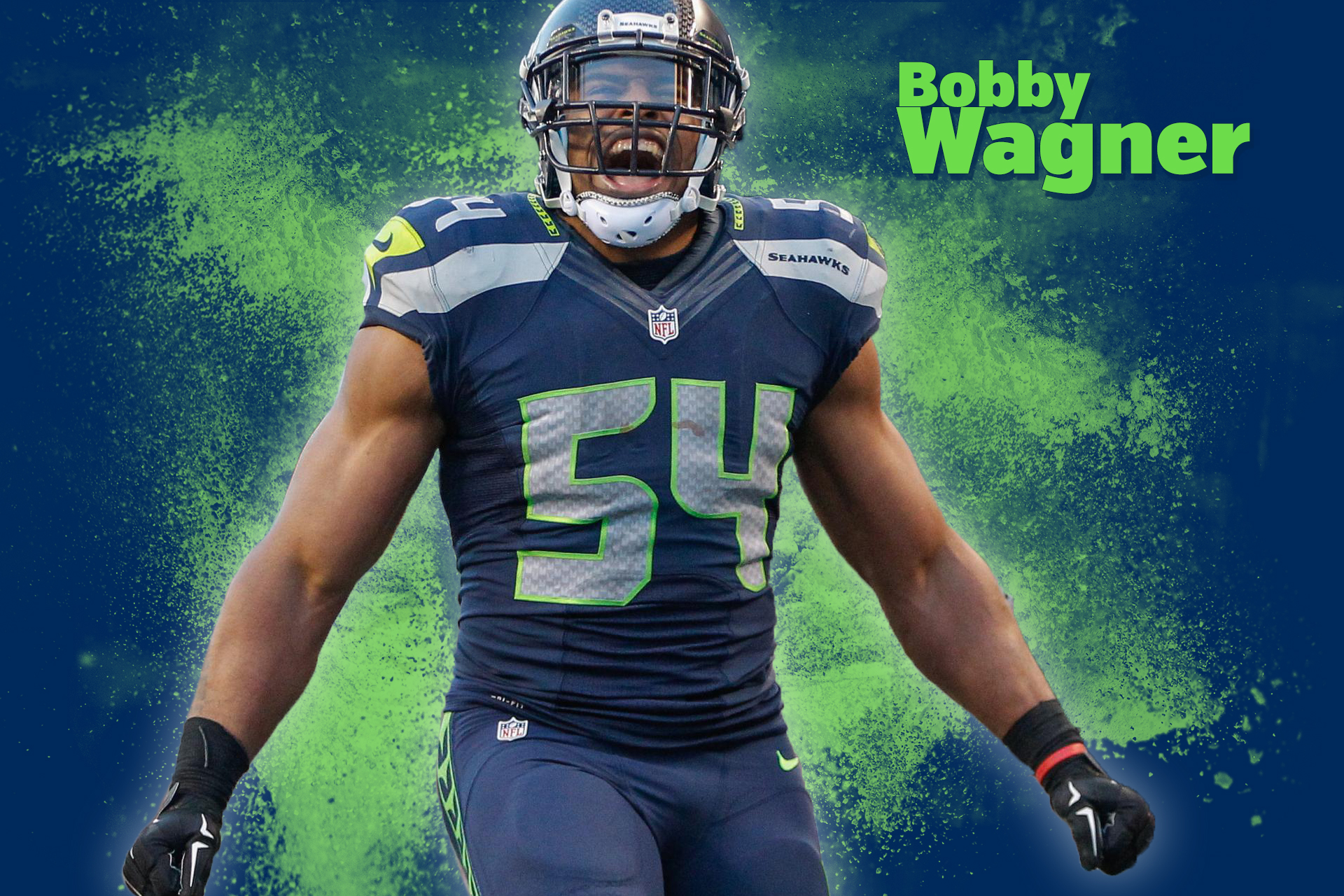The image features a dynamic portrait of an American football player, clearly identified as Bobby Wagner by the vivid yellow text in the upper right-hand corner. Wagner, a black man wearing a Seattle Seahawks jersey, stands centrally in the frame. He is adorned in the team's colors with a medium blue jersey featuring his number, 54, highlighted in light green. His uniform is complete with matching medium blue pants, black gloves, and a Seahawks helmet. Wagner's intense expression—mouth wide open and hands outstretched—suggests a powerful burst of energy, seemingly captured in a moment of exuberant scream or battle cry. The background is a visually striking mix, dominated by a deep Seahawks blue with an energetic explosion of light green, yellow, and orange paint splatters, adding a textured, artistic feel to the image. The player's figure has a subtle, semi-transparent shimmer, hinting at digital cropping techniques used to isolate him from the original context.